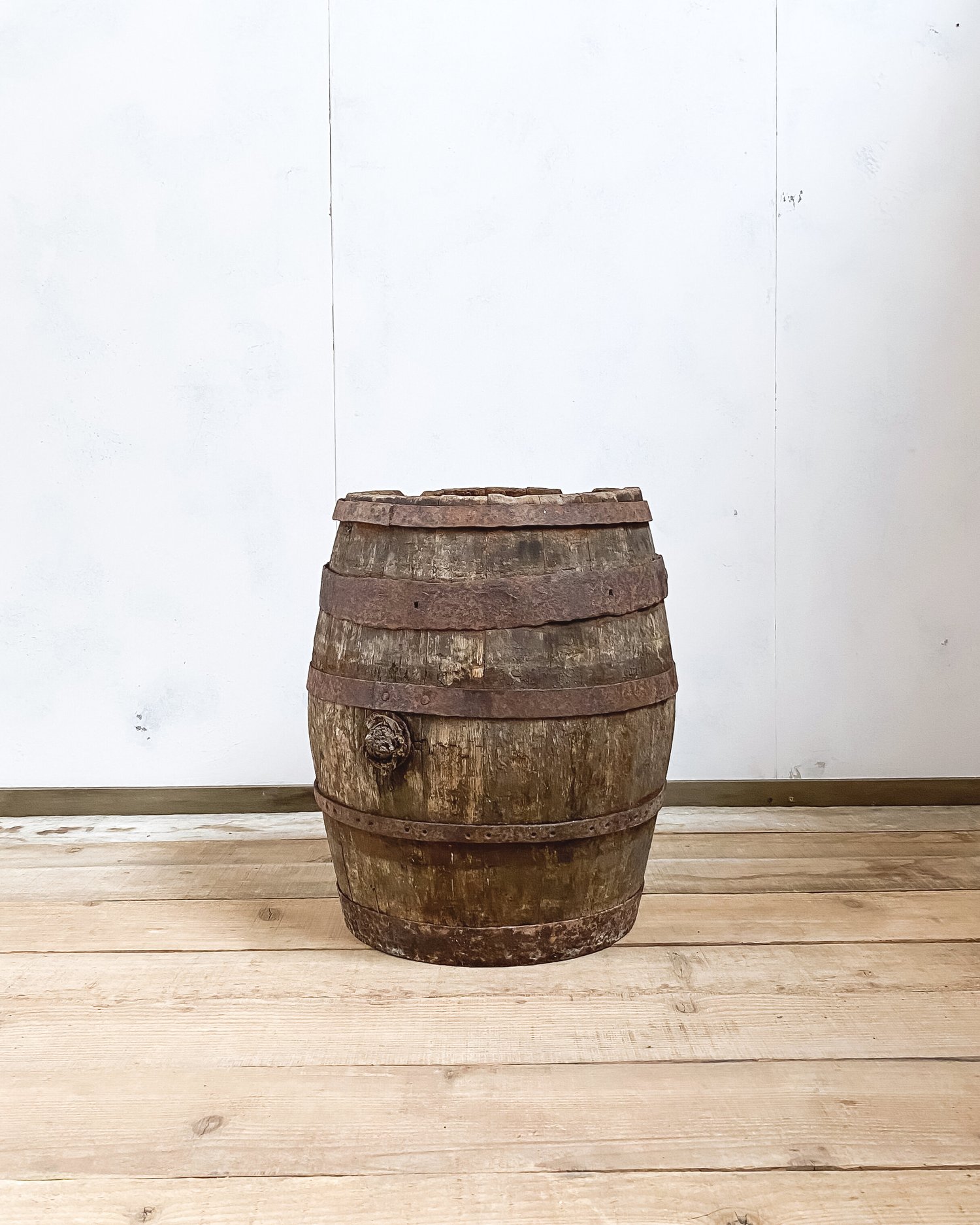This vertical, rectangular photograph depicts a weathered wooden barrel placed on a light-colored, natural wooden floor. The floor appears unfinished and rough, composed of raw wooden planks, enhancing the rustic appeal of the scene. The wall behind the barrel is painted white and consists of large panels with well-defined grooves between them. 

The barrel, aged and showing signs of significant wear, stands tall, accentuated by five rusted metal straps wrapped around it, which have lost their metallic sheen and turned a deep brown due to rust. The wood of the barrel appears aged and somewhat dilapidated, possibly waterlogged with the bunghole visibly rotted. The overall scene evokes a sense of antiquity and rugged charm.